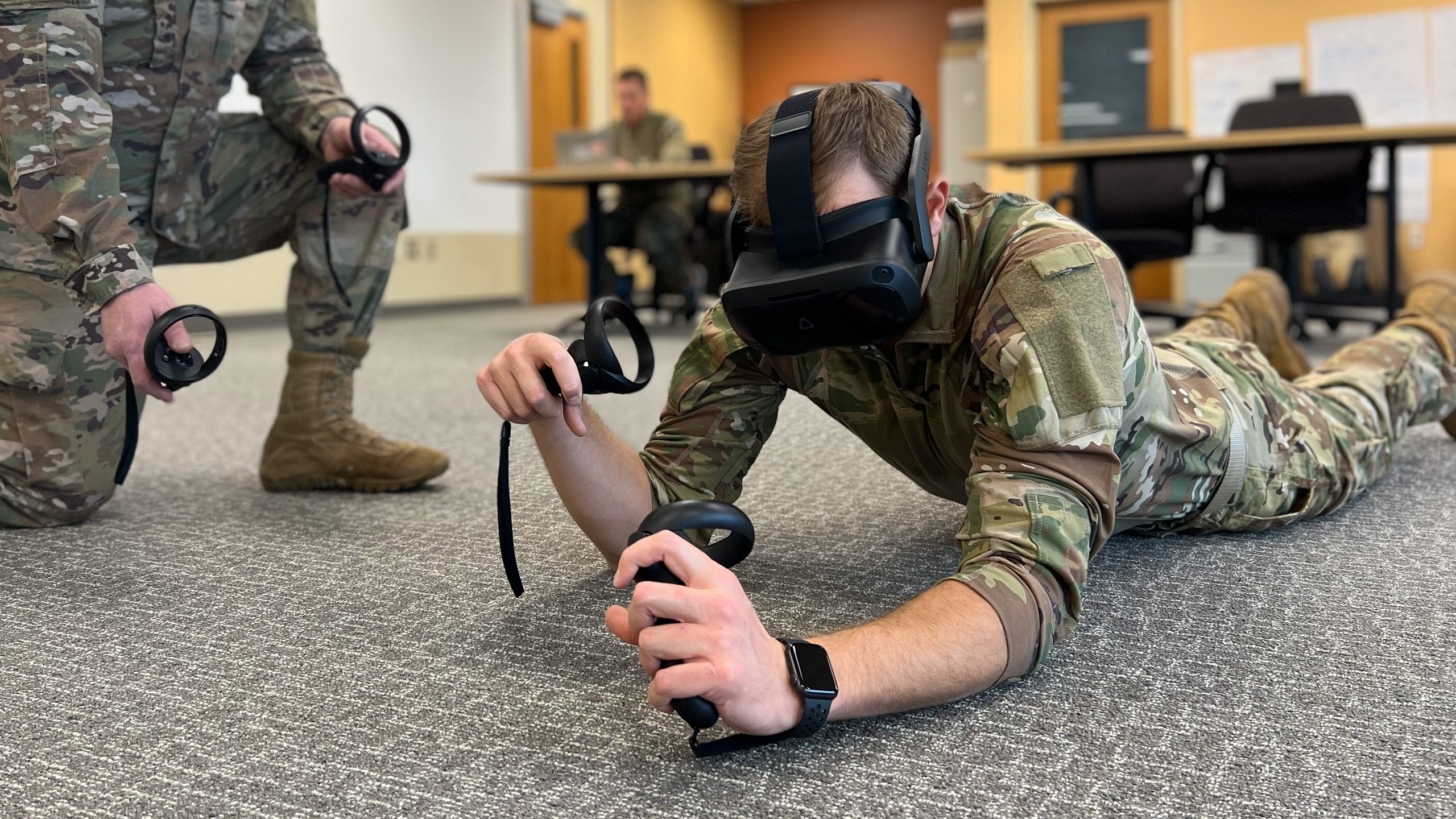In the image, three men in camouflage soldier uniforms are inside a room with a grey carpet patterned with white squares. The main focus is on one man lying on his stomach, his elbows propping him up. He is wearing black, box-shaped virtual reality goggles and holding two black controllers with circular grips. A black watch is strapped to his left waist. To his left lies another soldier, also on the floor, holding similar controllers. In the upper left corner of the image, a third soldier is kneeling down on one knee, his elbow resting on the other knee, partially cropped from the frame. In the background, a blurred soldier sits at a desk using a laptop. The room also features several tables, chairs, and doors, contributing to an office-like setting. The primary colors in the picture are green, brown, black, grey, and white.